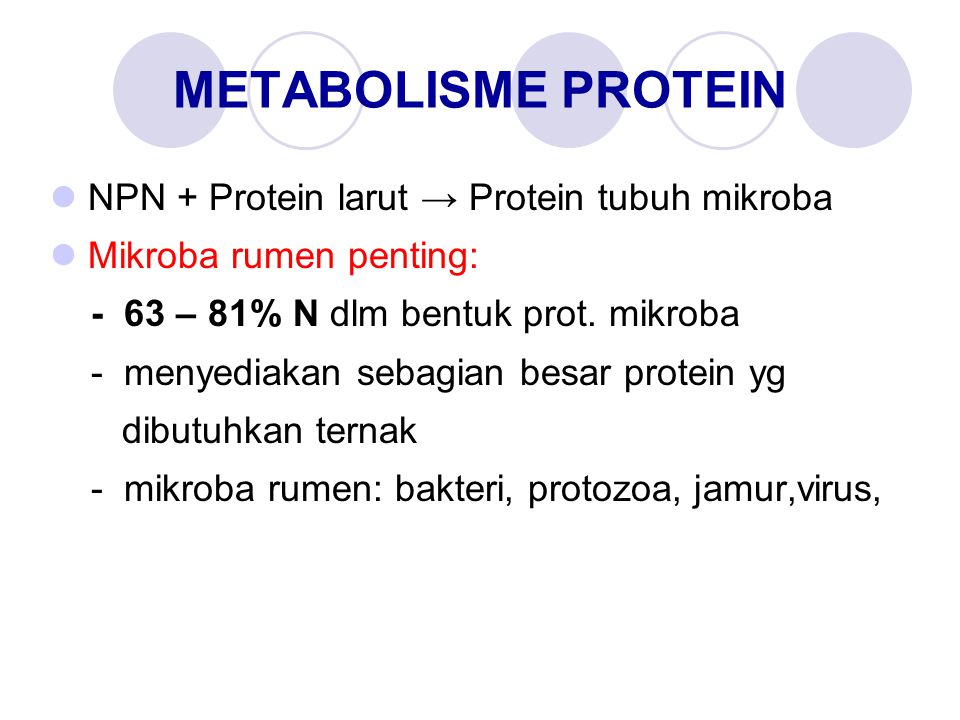The image depicts a presentation slide titled "Metabolizable Protein" in a dark purple-blue font, with the title positioned over a series of circles in varying shades of purple and white, likely symbolizing proteins. The slide contains two primary bullet points, both marked with purple-colored bullet symbols. The first bullet point, in black text, reads "MPN plus protein laureate, protein tuba, microba." The second bullet point, in red text, states "microba rumen pentate" and is elaborated upon with three sub-bullets indicated by dashes, discussing topics such as "important rumen microbes," "63 to 81% N protein form microbes," and the types of microbes which include "bacteria, protozoa, fungi, viruses." The background is white, and the overall layout appears to support a discussion on the significant role of microbe-derived proteins in livestock nutrition.